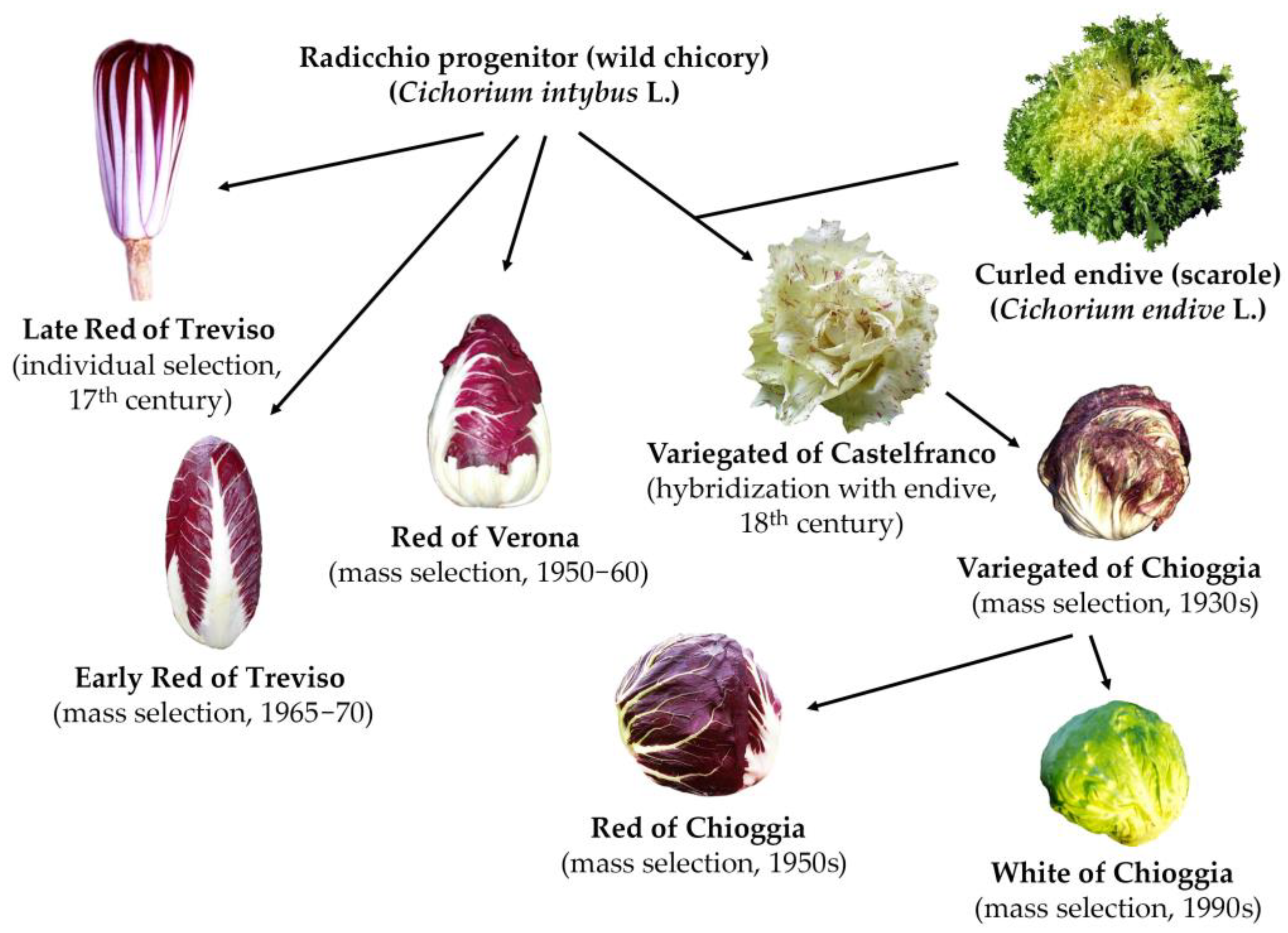The image displays a detailed botanical chart of various parts of a radicchio or wild chicory plant, scientifically named Cichorium intybus. Each part is meticulously labeled with black text and arrows against a white background. Dominating the top of the image is the title "Radicchio Progenitor" followed by "Wild Chicory" and its Latin name, "Cichorium intybus."

On the left side, detailed annotations describe "Late Red of Treviso," an individual selection from the 17th century featuring a red and white elongated vegetable. Just below it is the "Early Red of Treviso," a mass selection from 1965-70, also a red and white elongated variety.

Centrally, the image highlights the "Red of Verona," another red and white vegetable, a mass selection from the 1950-60 period. The bottom center of the chart showcases the "Red of Chioggia," a selection from the 1950s.

Moving to the right side, the image depicts the "Variegated Castelfranco," an 18th-century hybridization with endive. Above this is the "Curled Endive," also known as "Scarole" or "Chicorium Endive," marked as the Latin name. The "Variegated of Chicogia," a mass selection from the 1930s, occupies the right center, while the "White of Chicogia," a mass selection from the 1990s, is featured at the bottom right.

The image is a comprehensive representation of chicory-related plants and their historical descendance, focusing on the variations in color and form, particularly the intermingling of purple, white, and green structures.